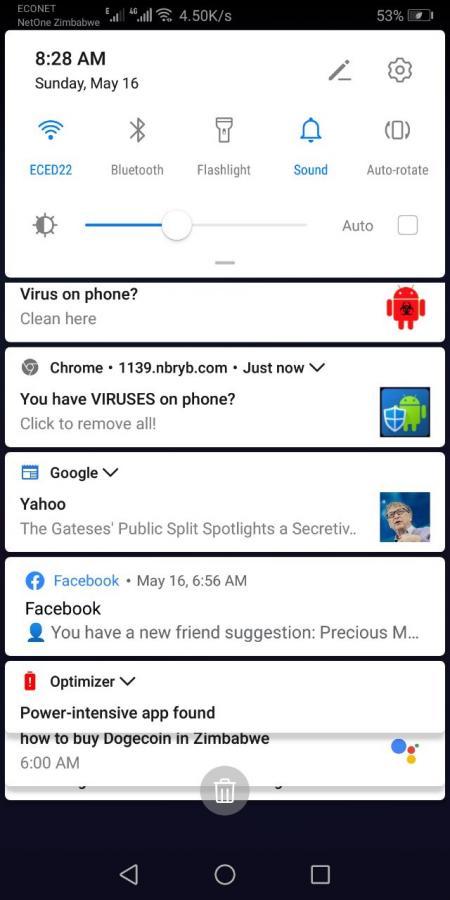Screenshot of Mobile Notifications on a Black Background: 
The mobile device screenshot displays various notifications layered on top of a black background, with each notification framed in a white box with slightly rounded corners. The background peeks through slightly between each notification, emphasizing their separation.

1. **Suspicious Notification Warning**: At the top notification, black text urgently states, "Virus on phone." Below this, in light gray text, it prompts, "clean here." To the right, a red Android icon features a black nuclear waste symbol, signifying a potential threat.

2. **Chrome Notification**: Directly underneath, a notification from Chrome is identified by a gray Chrome logo. The black text reads, "1139.nbryb.com," followed by a dot and "just now" in light gray, with a downward arrow indicating additional details. Bold black text alerts, "you have viruses on phone," followed by a light gray instruction, "click to remove all!" On the far right, a blue square houses a green Android icon paired with a blue shield outlined in white, signaling security concerns.

3. **Google Calendar Update**: Below the Chrome notification, a blue calendar icon symbolizes an update from Google, indicated in bold text with a downward arrow for more information. It is followed by "Yahoo" in black text and then light gray text that reads, "The Gates is public split," followed by "Spotlight's a secretive dot." To the right, a photograph of Bill Gates against a blue background adds a visual cue to the news.

4. **Facebook Notification**: The final notification features a round Facebook logo in blue, with the word "Facebook" also in blue. The light gray text notes the timestamp, "May 16th, 6:56 am."

Each notification provides distinct visual and textual cues, drawing attention to various alerts and updates, effectively leveraging icons and color codes for quick identification of their respective sources and urgency.